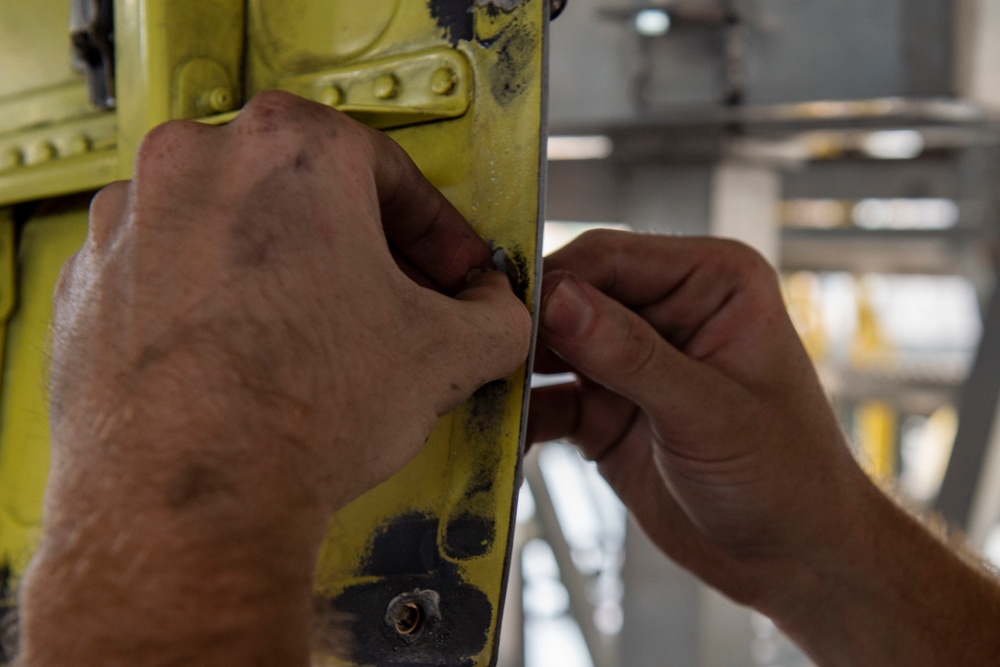In this detailed color photograph, we observe a close-up of a man's hands as he works with a small object, likely a screw or fastener, on a thin, yellow-painted metal surface. His left hand, prominently positioned on the left side of the image, is shown from the back. The skin on this hand is fairly light and adorned with dark hair on the wrist and hand. He grasps the screw delicately between his thumb and index finger.

On the opposite side of the yellow metal, his right hand is partially visible, with a clear view of his thumbnail, indicating that he is holding the metal steady. The object being worked on, along with the purpose of the task, remains ambiguous due to the limited view of the metal piece.

The blurred background on the right side of the photograph suggests that the setting could be the interior of a commercial building, possibly a store or a lobby with a glass door, though the exact details are indiscernible due to the significant out-of-focus effect.